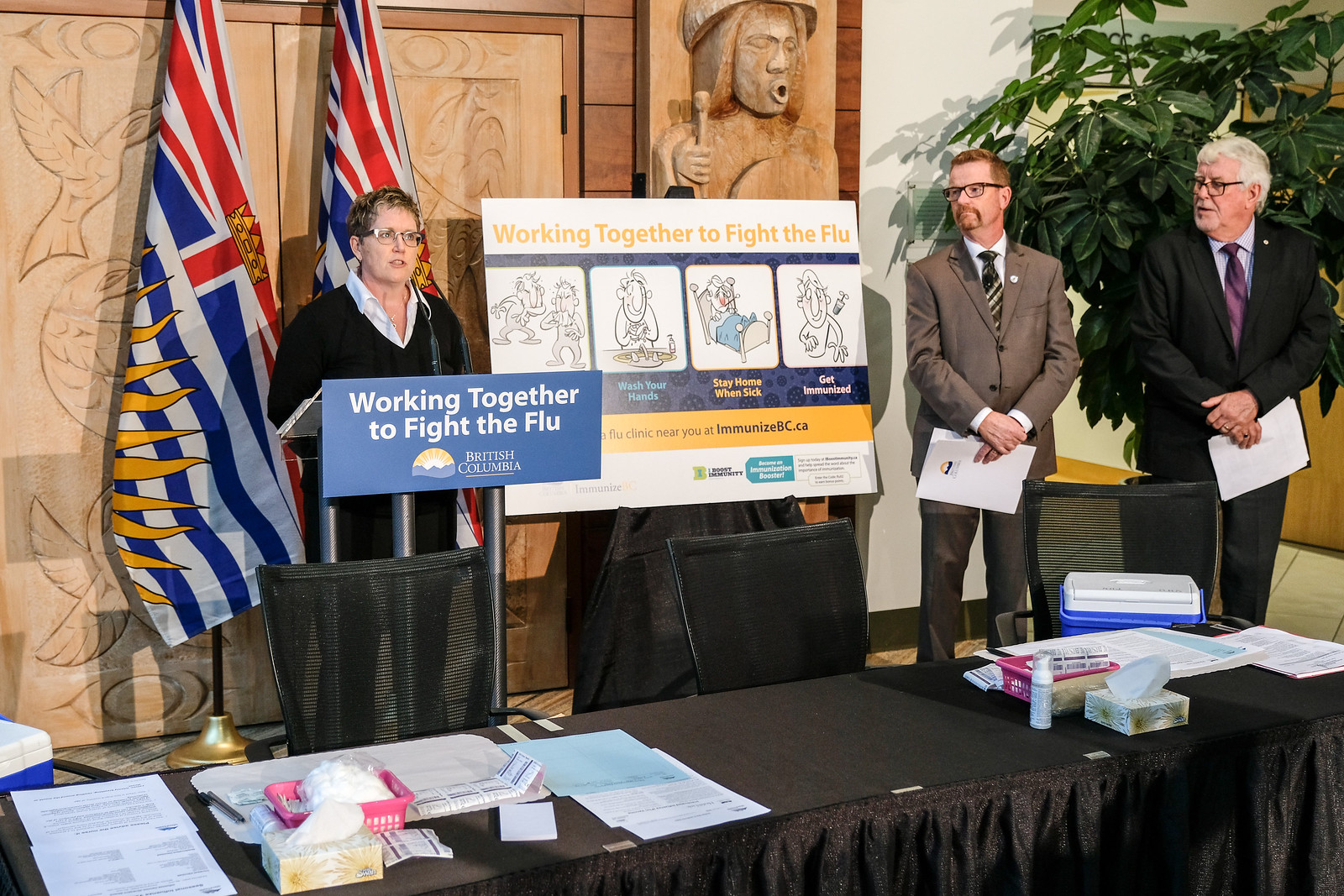Three individuals are positioned behind a sleek black desk. Starting from the right, a man with black glasses gazes to his left. He is a white male, dressed in a sophisticated black suit paired with a purple shirt and a dark purple tie. His hands are clasped over his stomach, holding some papers that hang downward.

Next to him, moving leftwards, stands another man, who faces front but turns his head slightly to the left. He is clad in a brown suit, complemented by a white shirt and a green tie. He also wears black glasses, sports a goatee, and has light brown hair. His hands are similarly positioned, clasped together over his stomach, clutching papers.

To their left is a white rectangular display board with the bold inscription "Working Together to Fight the Flu" at the top. Below this title, four segmented boxes contain black text focusing on the importance of flu vaccination.

Furthest to the left, a woman stands behind a podium. She is a Caucasian with short brown hair highlighted with lighter streaks and she wears black glasses. Her attire consists of a dark suit over a blue shirt. The podium displays a blue sign stating "Working Together to Fight the Flu of British Columbia." Behind her, two flags with red, white, blue, and some yellow elements hang against the wall. A wooden carving of a man with closed eyes, a round gaping mouth, and holding a stick in his left hand is mounted centrally above the scene.

The elongated black table in the foreground is littered with various items, including scattered papers, a pink box with a white substance, a tissue box, and a white bottle with a silver cap. Mesh-backed black chairs are arranged behind the table. In the bottom right corner, a blue-colored ice chest with a white lid is visible. Beyond the man on the right, a large green bush with broad leaves adds a touch of nature to the setting.